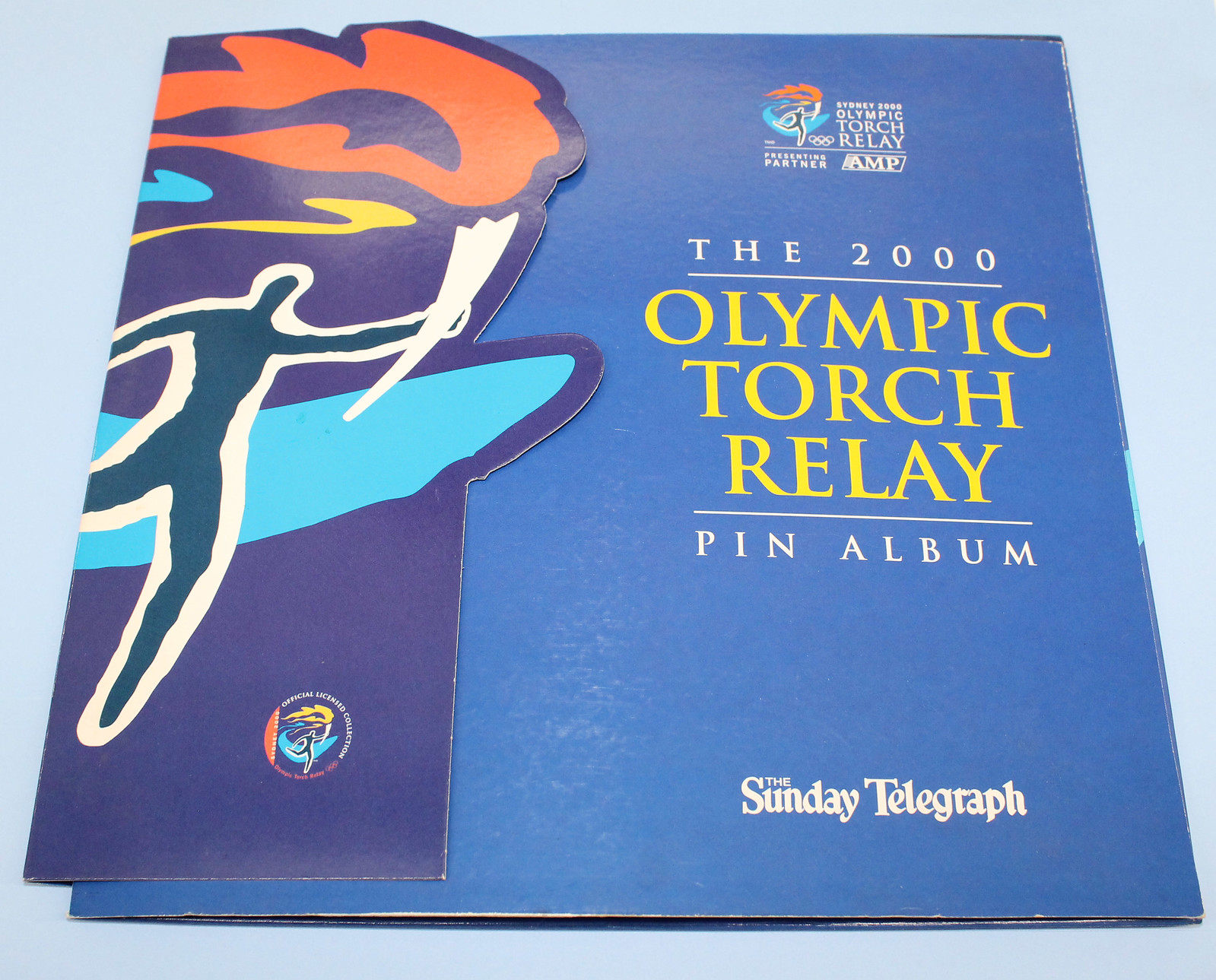This detailed caption describes a historic piece of Olympic memorabilia, the Sydney 2000 Olympic Torch Relay Pin Album, which was a promotional item associated with the Sunday Telegraph and Presenting Partner AMP. The album's cover is predominantly blue with accents of blue, yellow, white, and orange, lending it a unique and visually striking appearance. 

On the left side of the album is a cardboard flap that covers more than a quarter of the front. This flap features an artistic silhouette of a person carrying a long Olympic torch. The torch's flame is depicted in a stylized design with flowing red, yellow, and blue elements extending backward. The artwork not only provides visual appeal but also incorporates a cut-out design, following the contours of the silhouette and flame.

Central to the album cover are several key inscriptions in distinct color schemes: "Sydney 2000 Olympic Torch Relay" in yellow lettering, "The 2000 Olympic Torch Relay Pin Album" in white, and "The Sunday Telegraph" at the bottom, also in white. Additionally, a logo representative of the 2000 Olympic Games is prominently displayed, featuring a running figure holding a torch with orange flames and a blue swirl surrounding them. The album is placed on a blue-hued table, complementing the overall color theme of the cover, making this a vibrant piece of memorabilia from the 2000 Olympics.